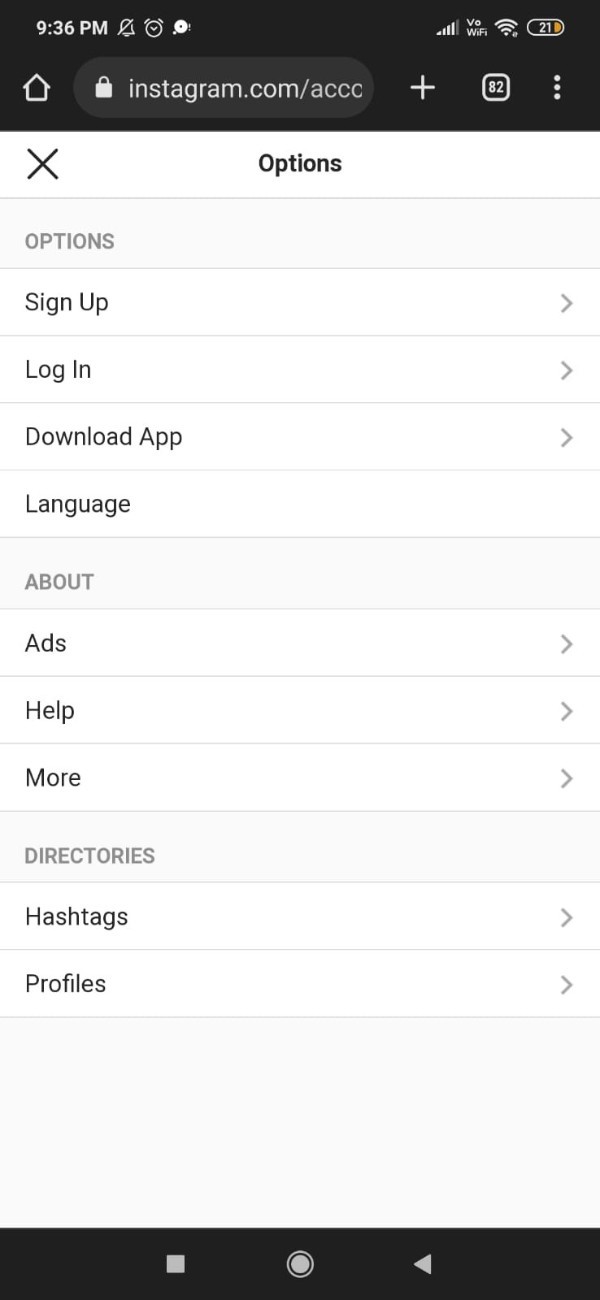The image depicts a screenshot taken from a mobile device showing the Instagram mobile website. The URL visible in the search bar begins with "instagram.com/ACC" but is partially obscured. The page displayed is the account options interface, labeled clearly as "Options" at the top.

The interface contains several sections with clickable links. The first section includes options such as "Sign Up," "Log In," "Download App," and "Language." Below this, there is an "About" section featuring choices like "Ads," "Help," and "More." Lastly, there is a "Directories" section listing "Hashtags" and "Profiles" for navigation.

The design of the website features a clean, white background with black text for clear readability. At the bottom of the screenshot, there is a black navigation bar with three white icons: a square, a circle, and an arrow pointing left. These icons likely correspond to various navigation functions such as back, home, and possibly other site-specific actions.